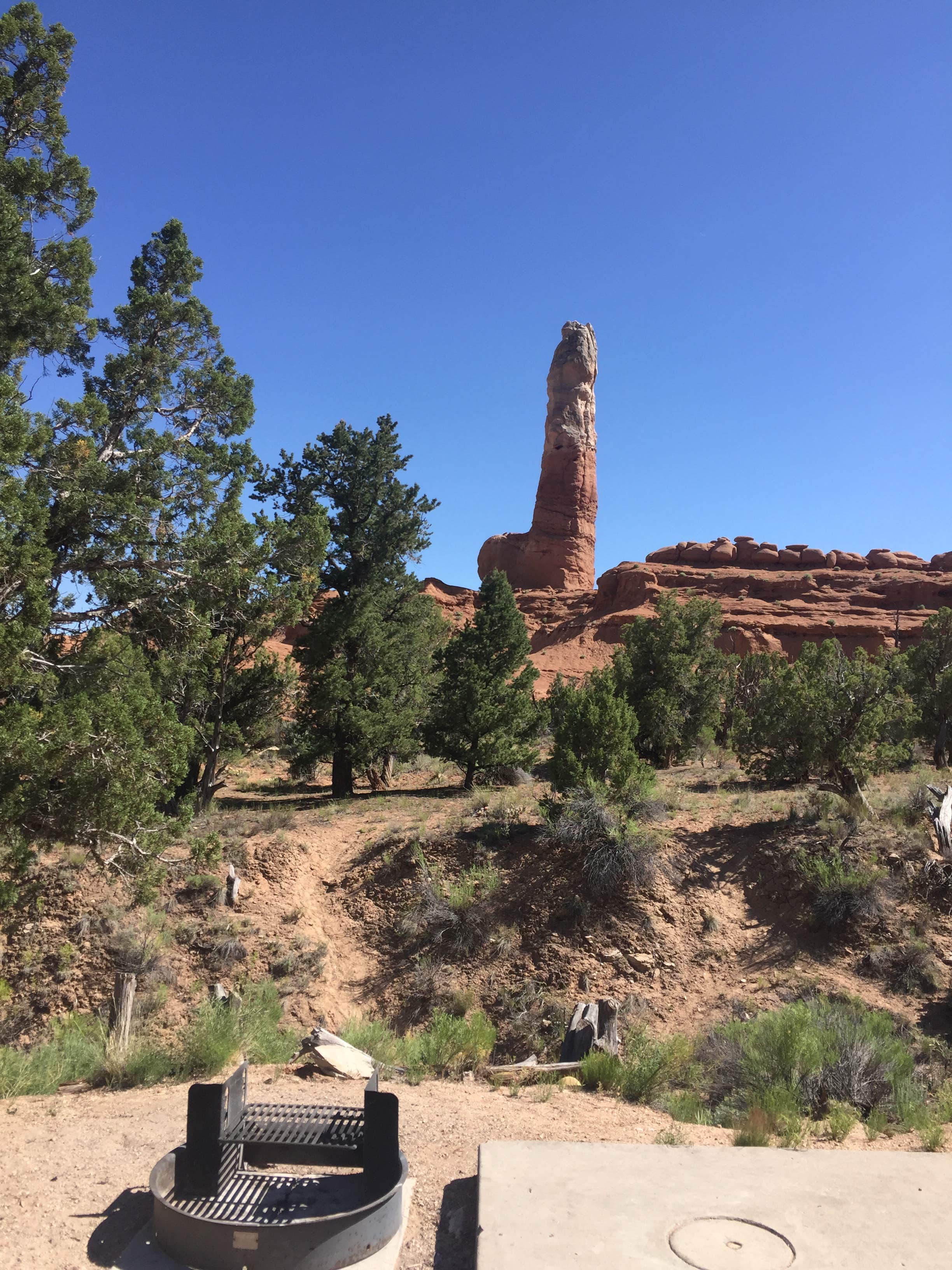The photograph depicts a deserted camping ground set in a dusty, arid desert environment that could be Arizona or Australia. Dominating the foreground is an open barbecue grill with two separate platforms. Close to the barbecue, there is a square metal platform and various camping objects scattered around. A well-trodden dirt trail starts here, meandering through sparse shrubby vegetation and green pine trees toward a stunning background. The landscape features a rugged reddish rock formation, which includes a distinctive tall, cylindrical rock. This formation is marked by a base of red ochre earth and a white-capped top section, accompanied by flatter, horizontally-layered rocks. The entire scene is bathed in bright sunlight under a cloudless blue sky, emphasizing the barren, sun-soaked atmosphere.